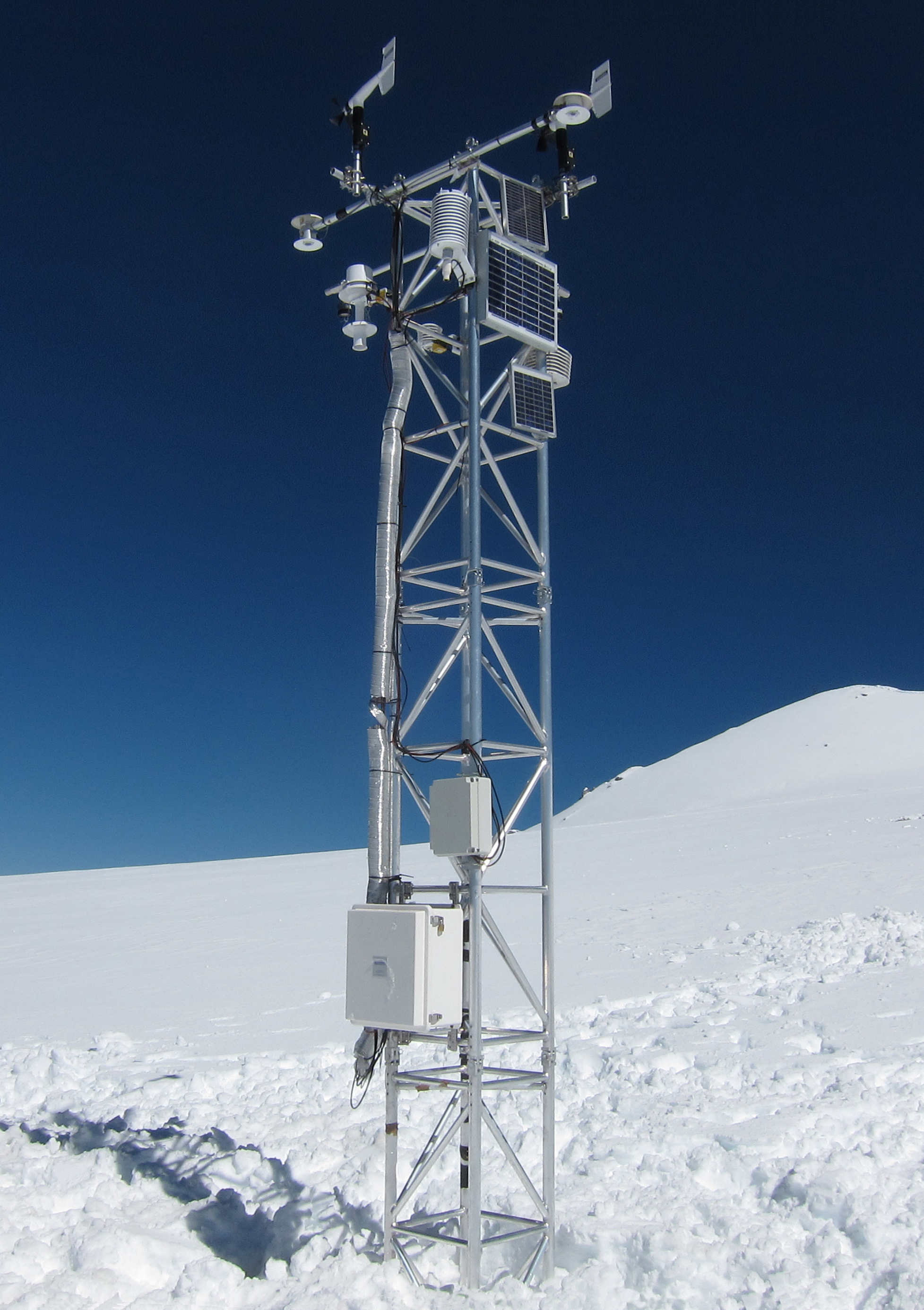This photograph showcases a tall, metal structure likely used for weather monitoring or scientific purposes, situated in a cold, snow-covered environment. The structure, made of steel beams, features a small electronic power box at the base and several small solar panels at the top. Additional elements include cylindrical coils and various electrical boxes and wires. The ground is completely covered in snow, with the foreground appearing disturbed, possibly from human activity. In the background, the landscape is mainly flat, with some mounds or hills of snow. The sky is remarkably clear and transitions from a light blue near the horizon to a darker blue higher up, enhancing the stark, isolated beauty of the scene.